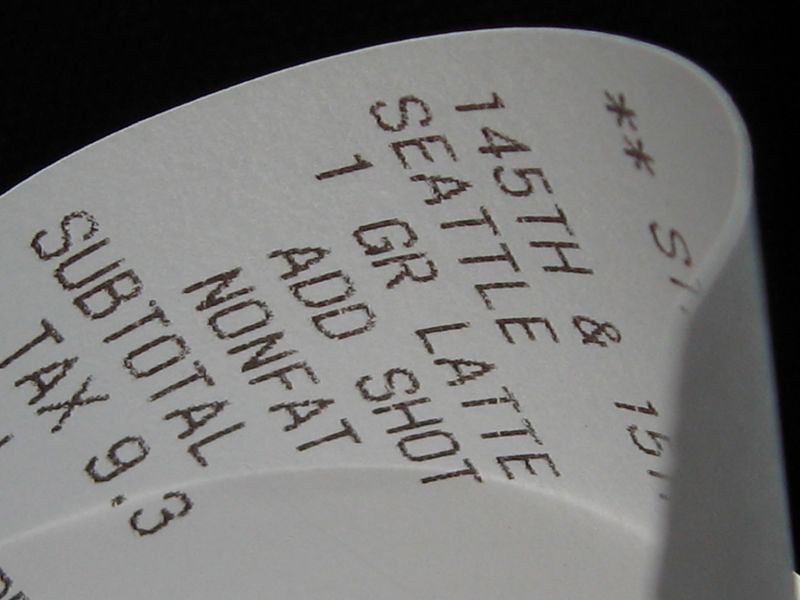A partially folded Starbucks receipt is displayed in the image. The visible portion begins with the letters "ST," suggesting it’s from a Starbucks location. The rest of the establishment's name is obscured by a fold in the paper. The address mentioned on the receipt indicates the location is at the intersection of 145th Street and 15th Avenue in Seattle. The detailed order lists one grande latte with an additional shot and non-fat milk. Though the subtotal amount is obscured due to the paper’s fold, the tax rate is clearly visible at 9.3%, likely representing the local sales tax. The receipt is white with black printed text, common for point-of-sale receipts.